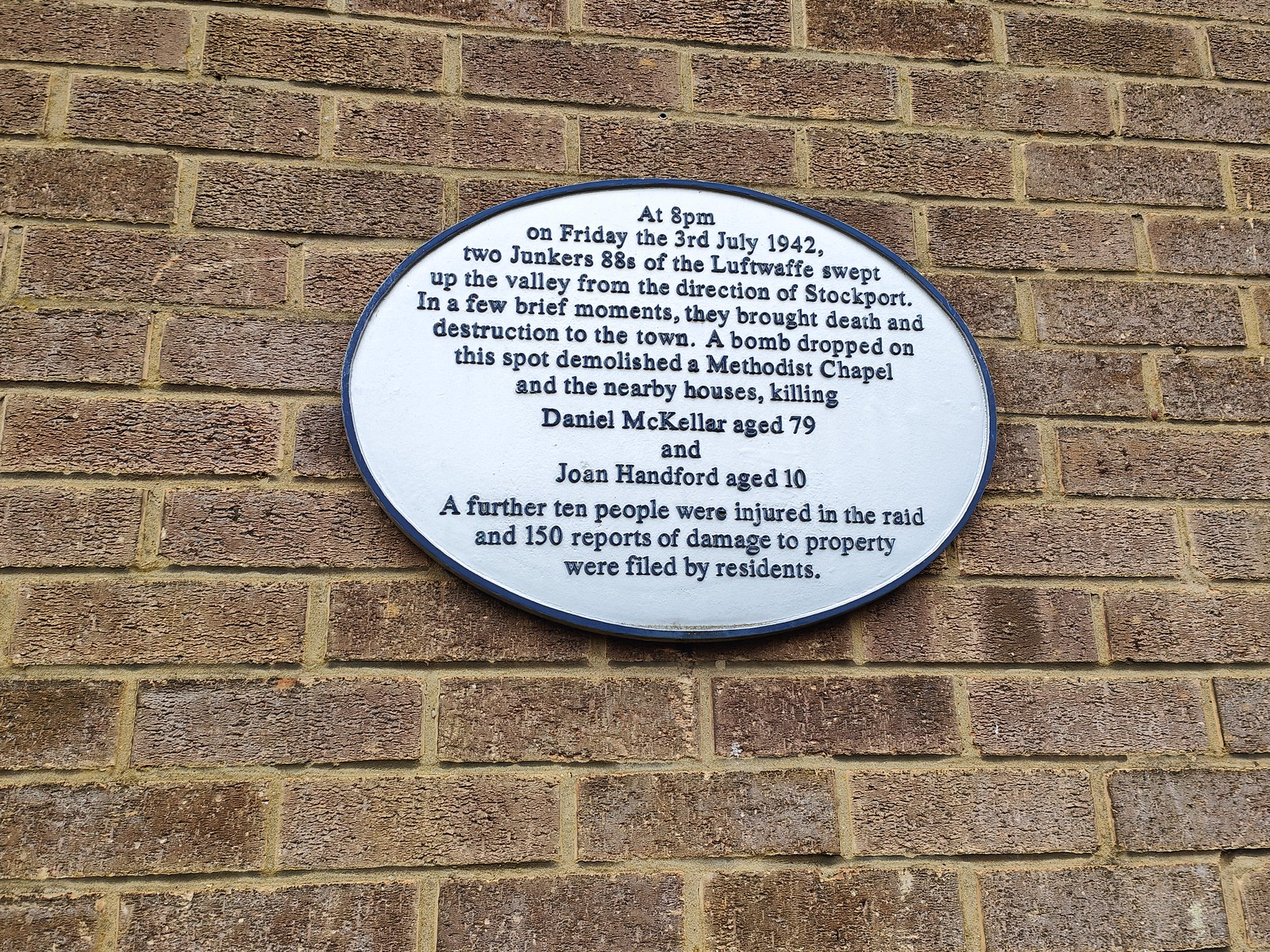The photograph, taken outdoors during the daytime, features a predominantly square, slightly rectangular image of a reddish-brown brick wall with lighter tan grout. Central to the photo is an oval plaque with a navy blue outer ring and a white background featuring raised blue lettering. The plaque text details the tragic events that occurred at 8 p.m. on Friday, July 3, 1942, when two Junkers 88 bombers of the Luftwaffe swept up the valley from Stockport, bringing death and destruction. A bomb dropped at this spot demolished a Methodist chapel and nearby houses, killing Daniel McKellar, aged 79, and Joan Hadfield, aged 10. Additionally, 10 people were injured, and residents filed 150 reports of property damage.